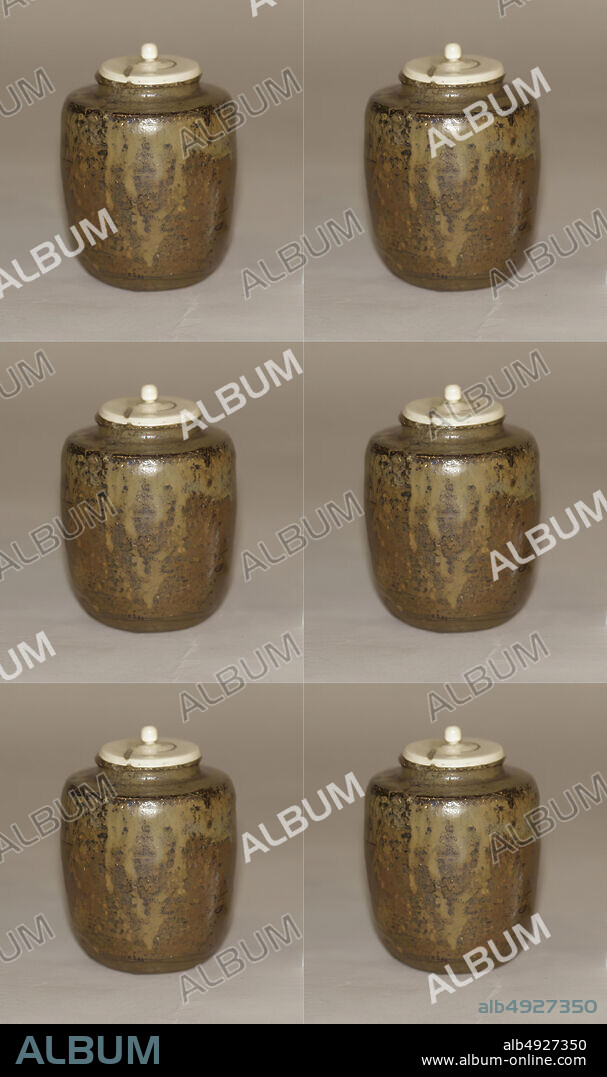The photograph is a vertically oriented image featuring six identical squares, each containing the same realistic depiction of a brown, tan-streaked ceramic jar with a white lid and a small round knob. The jars, which could be urns or antique crocks, are arranged in two columns and three rows. A repeated watermark of the word "ALBUM" in white overlays the entire image, suggesting a copyright protection method often used for digital content. At the bottom of the photograph, a black bar displays the text "ALBUM" in blue font, accompanied by a reference number "ALB 4927350" and the website "www.album-online.com," indicating that this could be an advertisement for the jars or a photo printout used for business purposes.